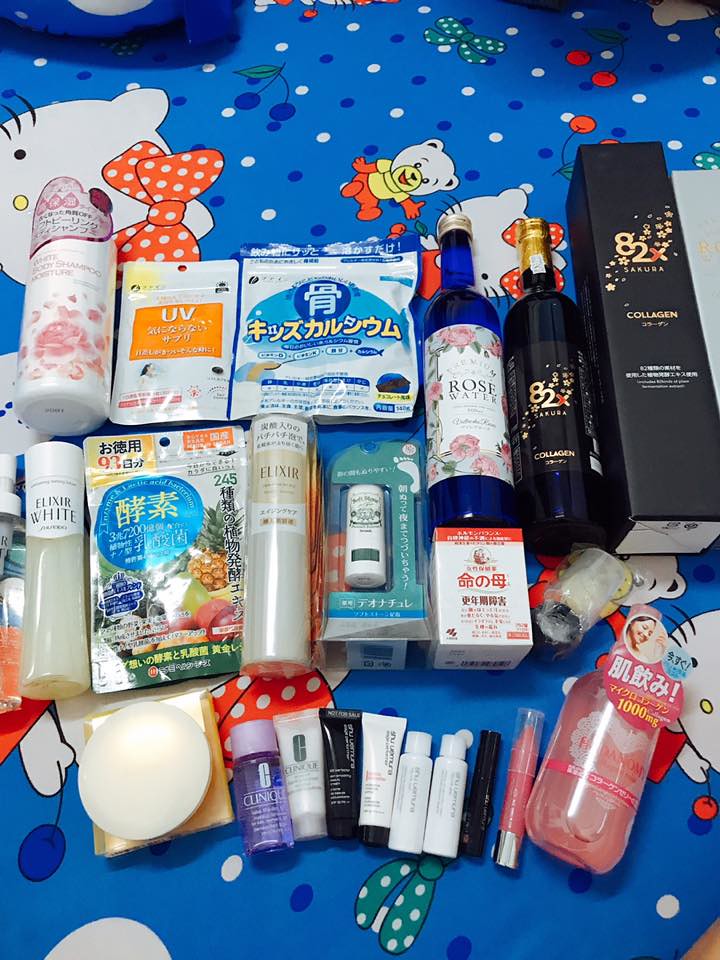Displayed on a blanket adorned with various Hello Kitty characters, including Hello Kitty herself sporting a green or orange polka-dotted bow, a little bear, cherries, and numerous small bows, is an assortment of Japanese-labeled products. Among these items is a black box containing a bottle labeled "collagen", as well as a blue glass bottle labeled "rose water". Additionally, there are two items from the brand Elixir and two from Clinique, suggesting they could be makeup or skincare products, each lying on their side. Also visible are a couple of pouches, though their contents remain unknown.